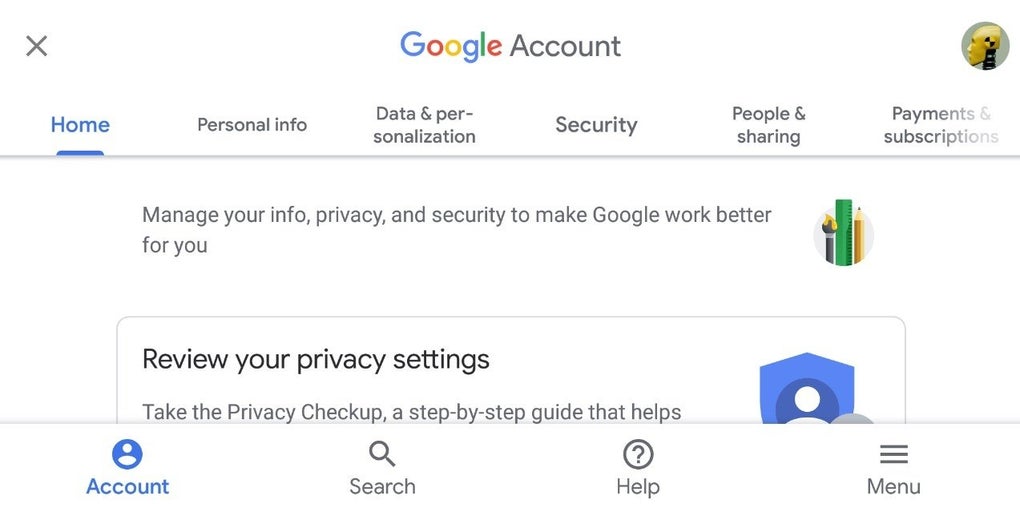The image showcases a Google Account settings page, featuring various categories for managing different aspects of the user's account. The categories listed prominently on the left-hand side include: 

- Home
- Personal Info
- Data and Personalization
- Security
- People and Sharing
- Payments and Subscriptions

Below these primary categories, users can also find options to manage their information and enhance their privacy and security settings with features like "Manage Your Info," "Privacy," and "Security to make Google work better for you." Further options include "Review Your Privacy Settings" and "Set The Privacy Checkup," a step-by-step guide designed to help users navigate their privacy options.

At the bottom of the page, additional navigation options include "Accounts," "Search," "Help," and "Menu," each represented by different colored icons: green, red, yellow, blue, and black, adding a visually organized touch to the interface.